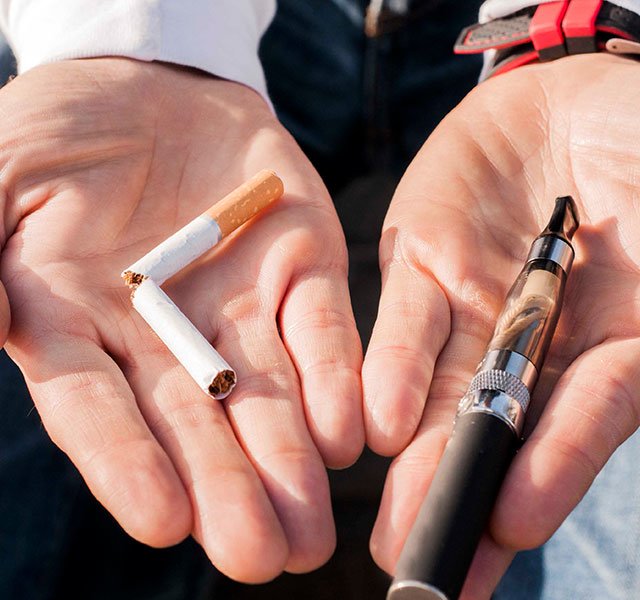A photograph captures a man standing on what appears to be a sidewalk, illuminated by sunlight coming from an angle, casting distinct shadows beneath the objects in his hands. The man's outstretched, palms-up hands are framed against the background, revealing a white dress shirt with sleeves that extend to his wrists and a black and red watch on his left wrist. In his right hand, held prominently in the center of his palm, is a broken cigarette with the white portion snapped and the brown filter still intact. In his left hand, he holds a black and chrome electronic vaping device with a small mouthpiece. The contrast between the intact vape pen and the broken cigarette suggests a visual commentary on the harmful effects of smoking. The man's skin is of a white complexion, and he is wearing black pants, adding to the sharp contrast and clarity brought out by the sunlight that highlights the contours and details of his hands and the objects they hold.